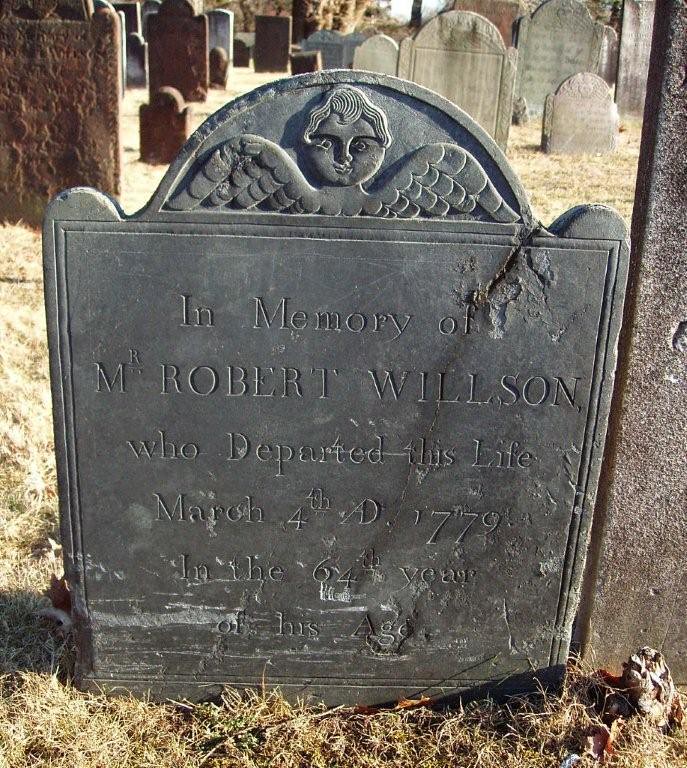In the foreground of this autumn or winter scene, an old graveyard lies with its weathered, raised headstones. The surrounding grass appears lifeless or dormant, contributing to the somber mood. The headstones, varying in age and color, number around 15 to 20 and stand as solemn reminders of the past. They appear almost ancient, bathed in a faded palette of hues that reflect their enduring presence. The main headstone commands attention with its dark gray patina and ornate etchings. Though aged and worn, one can still decipher its inscription: "In memory of Mr. Robert Wilson who departed his life March 4th, 1779 in the 64th year of his age." This striking monument, over 200 years old, encapsulates the passage of time and the persistence of memory.